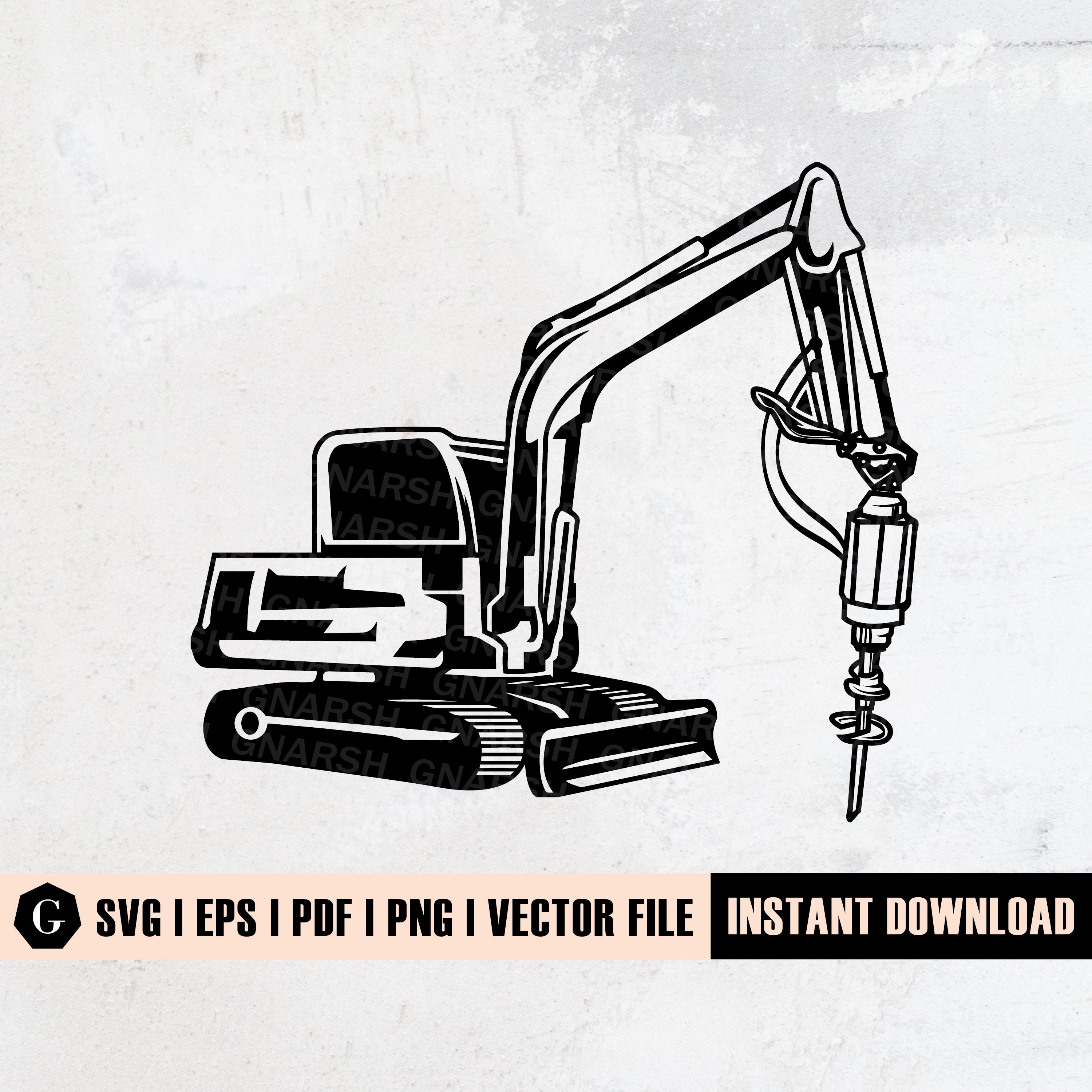The image depicts a high-contrast, black-and-white line art drawing of a large piece of heavy machinery with detailed features. Centered prominently, the machine consists of a main body on the left, equipped with rotating track tires reminiscent of a tank, and a shoveling scoop at the front. A cockpit area with blacked-out windows is visible on the body, while an articulating arm extends to the right, ending in a substantial drill bit or jackhammer facing downward. The background is textured in shades of white, gray, and ivory, adorned with repeated light gray watermarks reading "GNARSH." Below the image, a footer provides format options in black and peach tones: SVG1, EPS1, PDF1, PNG1 vector file. To the right of this list, within a black bar, 'Instant Download' is displayed in white lettering.